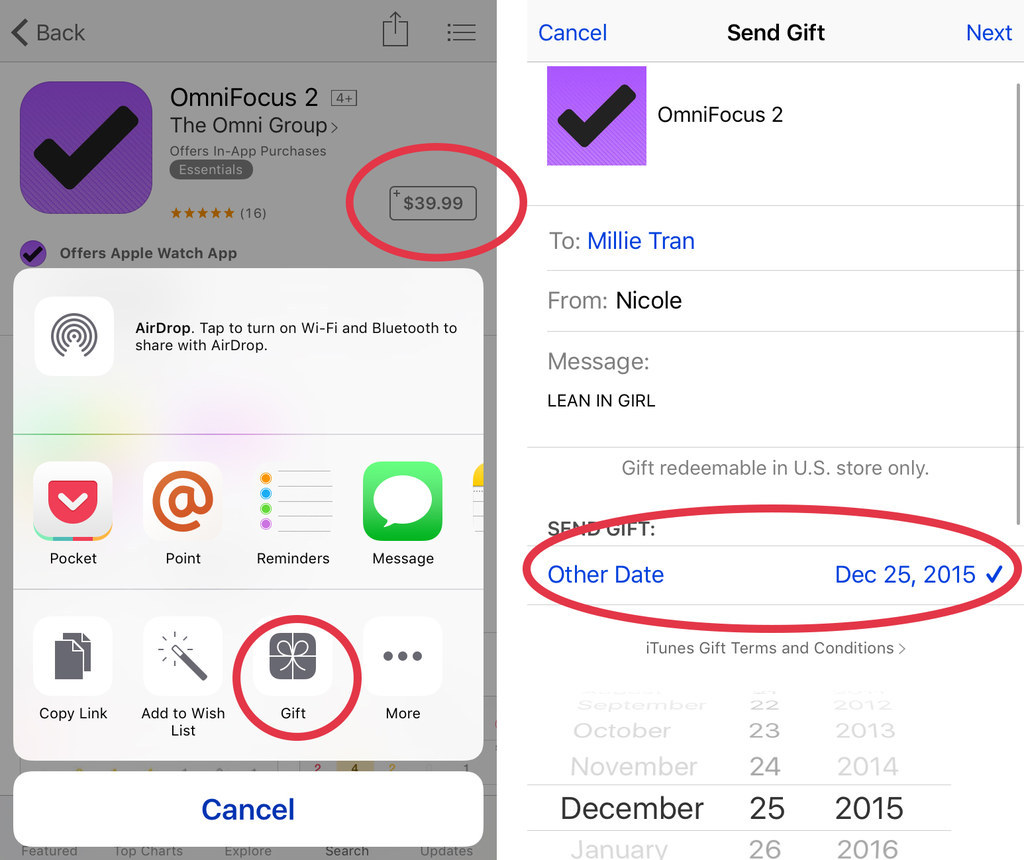The image consists of two cell phone screenshots placed side by side. The screenshot on the left displays the purchase details of the app "OmniFocus 2" from the Omni Group, with a red circle highlighting its price of $39.99. Additionally, there's a pop-up menu providing options such as copying the link, adding to a wishlist, and gifting the app. The "gift" option is represented by an icon resembling a present viewed from above, with the text "gift" underneath it, indicating that the app can be purchased as a gift for someone else.

The screenshot on the right shows that the app has indeed been gifted, with the gifting date marked as December 25th, 2015. It displays the recipient's and sender's information, along with a section where a personalized message can be included with the gift.